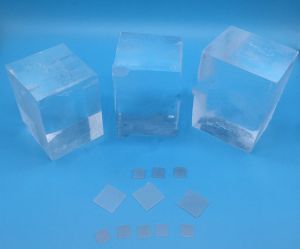The image depicts a collection of transparent, cube-like structures arranged on a light blue background. Dominating the back row are three large, gelatin-like cubes of varying sizes. The smallest cube on the left features a mysterious white reflection on its bottom right corner. The middle cube is slightly larger and has a noticeable chip on its top left corner. The largest cube on the right is perfectly formed with equal dimensions in height, width, and depth, and it appears to be the clearest of the three.

In front of these three prominent cubes, there are a series of smaller square sheets and blocks laid out in a structured arrangement. These smaller objects are organized in three distinct rows: the first row comprises three small squares, the second row consists of three larger squares touching corner to corner, and the final row includes five even smaller squares. The arrangement and material of these smaller squares suggest they might be off-cuts or related samples of the larger cubes. The meticulous layout on the light blue background adds a scientific or experimental aesthetic to the image.